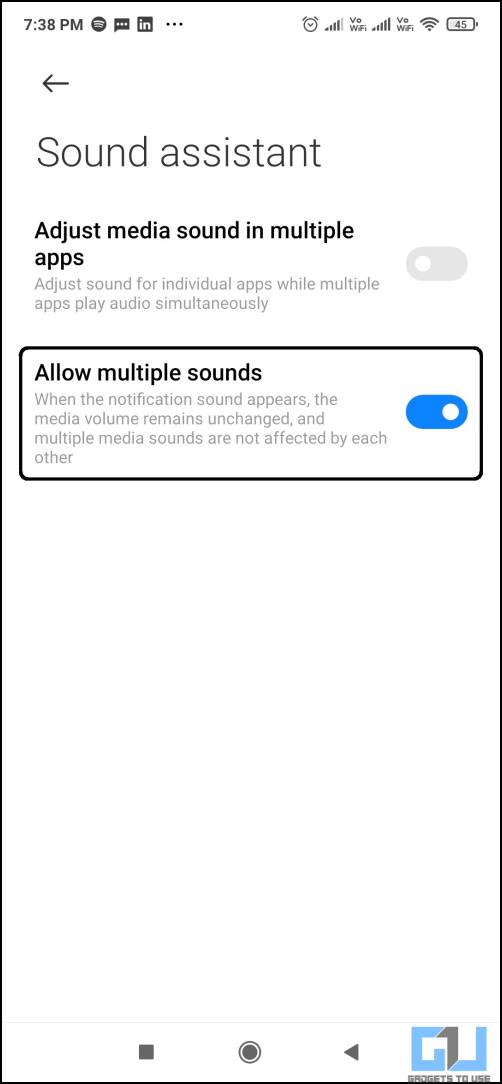In the provided image, there is a grey-outlined rectangle, with the timestamp "7:38 PM" displayed in the top left corner. Below the timestamp, there are several icons: a circle with white lines inside, a rectangular icon with a few dots, and a square marked with the letter "N." Adjacent to these is a row of three horizontal dots aligned side by side.

On the right side of the rectangle, the first icon appears to be a clock. Following this, there are lines of increasing length moving rightwards, interspersed with letters, ending with a Wi-Fi symbol and a battery icon displaying "45." 

Below these icons, a left-pointing arrow precedes the text "Sound Assistant." Directly underneath is the phrase "Adjust Media Sound in Multiple Apps," followed by additional grey text. Further down, there is a grey button with a white circle inside. The button sits within a black-outlined rectangle bearing the text "Allow Multiple Sounds," with more explanatory words beneath it. 

A blue button, also featuring a white circle, is positioned further down. A significant amount of blank space leads to the bottom of the image where there is a grey square, a grey-outlined circle with another grey circle inside, a grey triangle pointing to the upper right, and a dual-toned symbol that resembles the letters "GU" in blue and grey.